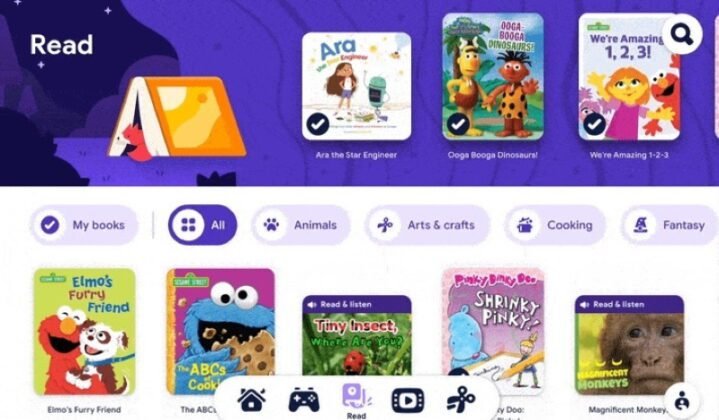Here is a detailed and cleaned-up descriptive caption for the image:

---

The image depicts a vibrant reading application designed for small children. The top left corner features the word "Read" in white font. The application's background is a deep purple, reminiscent of a nighttime sky adorned with stars, accompanied by silhouettes of mountains and trees. 

In the foreground, a red fox peeks out from the white opening of an orange and yellow tent. The tent, which also displays gold, light tan, and orange lines along with a sun illustration, stands out against the dark backdrop. Three books are prominently displayed next to the tent, each with a white check mark encased in a black circle beside them.

1. **"Ara the Star Engineer"** - This book features a little girl and a robot and has its title written on the tent.
2. **"Ooga Booga Dinosaurs"** - Depicts Bert and Ernie holding hands in what looks like a jungle setting.
3. **"We're Amazing 1, 2, 3!"** - Showcases another Sesame Street-themed cover.

Beneath the main display, various book categories are listed: "My Books," "All," "Animals," "Arts and Crafts," "Cooking," and "Fantasies." The section titled "My Books" includes "Sesame Street's Elmo's Furry Friend," showing Elmo hugging a small brown and white dog. 

A separator line follows, leading to titles such as "Sesame Street's The ABCs of Cookies," "Tiny Insects: Read and Listen," "Shrinky Pinky Boo," and "Magnificent Monkeys: Read and Listen."

At the bottom of the screen, icons illustrate different functionalities, including a house, a video game controller, a TV screen, and a pair of scissors. Currently, the "Read" option is highlighted in light purple.

---